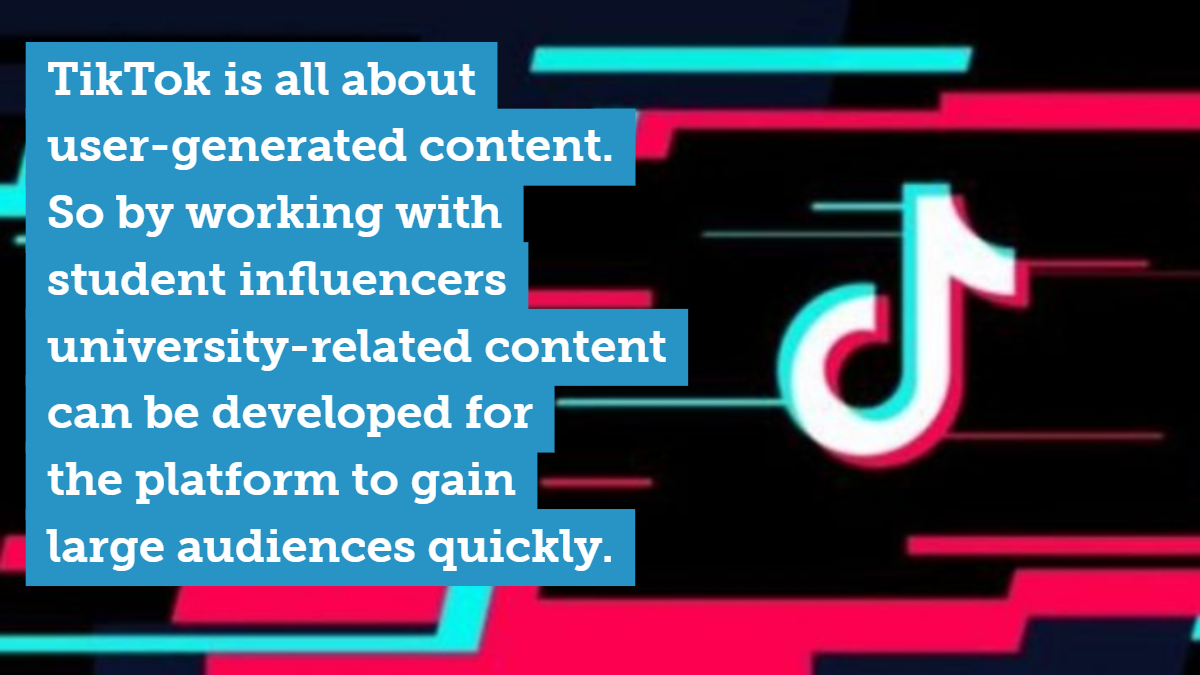The provided image is a screenshot set against a black background adorned with decorative accents in aqua and red. At the top of the image, there is a solid aqua bar, followed by a uniquely shaped red bar directly beneath it. Below this, lie two fine aqua lines. Continuing downward, there is a thicker red line, trailed by another fine aqua line. As we progress further, we encounter two fine red lines, succeeded by an additional fine red line. Near the bottom of the image, there are four distinct red shapes and a relatively bold aqua line. On the right side of the screenshot is the TikTok logo. To the left, there's a blue box containing white text that reads: "TikTok is all about user-generated content. So by working with student influencers, university-related content can be developed for the platform to gain large audiences quickly." This text occupies approximately half of the image.